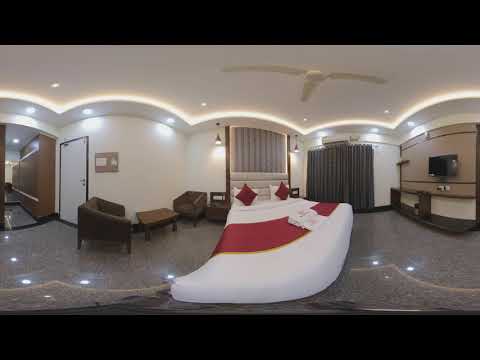This panoramic photograph of a bedroom captures all four walls of the room, showcasing its modern interior. The walls and ceiling are white, with a white, centrally located ceiling fan. The flooring appears to be highly reflective, gray-toned linoleum, sometimes described as marble-like. Along the left, there is an open doorway leading into a smaller seating area containing two small brown-gray chairs and a small table. Adjacent to this is another wall featuring a door. The main focal point, however, is a large bed against the central wall which features a high, white leather headboard. The bed is adorned with white linens, accented by a burgundy runner at the foot and a mix of burgundy and white decorative pillows at the head. On the right side of the room, gray curtains extend nearly the entire length of the wall, and a mounted TV with a console table beneath it is also visible. The room is also illuminated with white, reflective can lights around the wall's trim, adding to the elegant ambiance. The image itself has a unique, warped perspective, indicative of being taken with a 360-degree camera and laid flat, which gives a curvy and elongated appearance to the ceiling and bed.